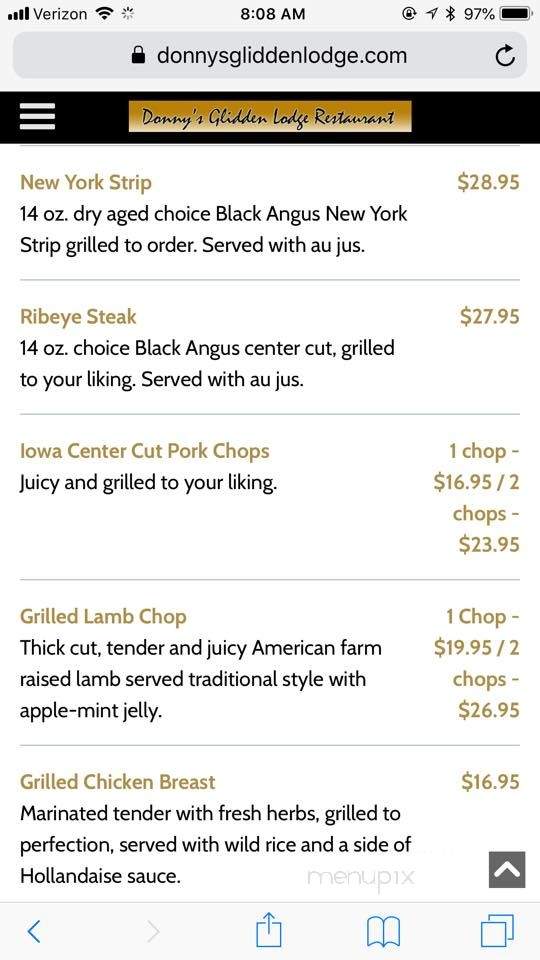**Detailed Caption:**

A screenshot captured from a cell phone displaying Donnie’s Glidden Lodge Restaurant website. The phone is connected to Verizon, showing four bars of signal strength. The Wi-Fi is on, Bluetooth is active, and the battery is at 97%. The time displayed is 8:08 AM. 

At the top of the screenshot, the browser's address bar is visible. Below it lies a black navigation bar on the website interface, featuring a hamburger menu icon on the left. Centrally positioned in gold lettering, it boldly reads "Donnie's Glidden Lodge Restaurant."

The menu section displayed includes detailed descriptions of various dishes and their prices:
- **New York Strip**: A 14-ounce dry-aged choice Black Angus New York strip steak grilled to order, priced at $28.95.
- **Ribeye Steak**: Listed at $27.95.
- **Iowa Center Cut Pork Chops**: One chop for $16.95, or two chops for $23.95.
- **Grilled Lamb Chop**: One chop for $19.95, or two chops for $26.95.
- **Grilled Chicken Breast**: Priced at $16.95.

At the bottom of the screen, the website's options are represented by icons: a square with an upward arrow (typically for sharing), a book (possibly for bookmarking), and two overlapping squares.